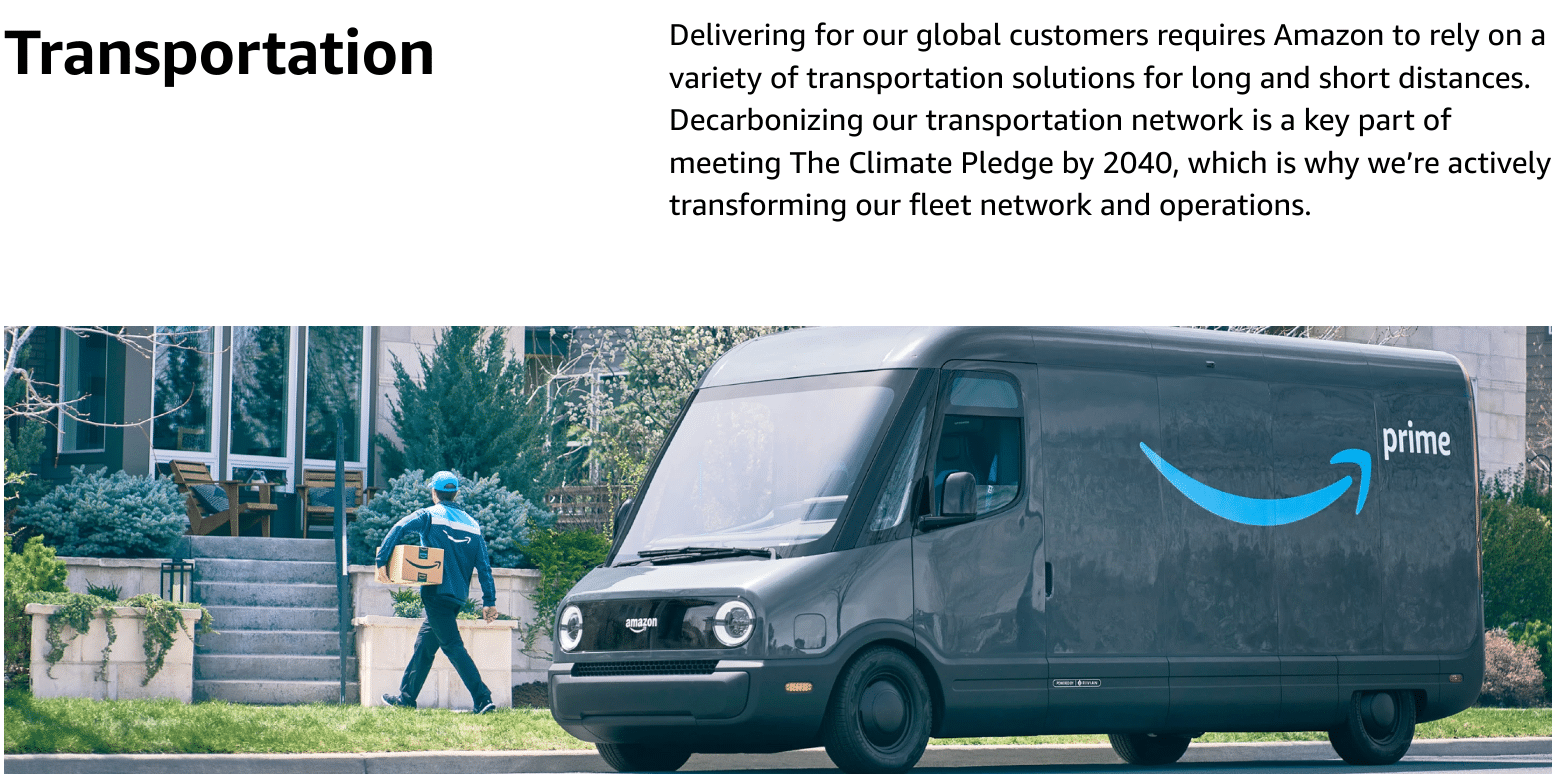This image captures a diverse narrative set against a crisp white background. On the upper left, bold dark gray text reads, "Transportation." Adjacent to it, in light gray text, a detailed message states: "Delivering for our global customers requires Amazon to rely on a variety of transportation solutions for long and short distances. Decarbonizing our transportation network is a key part of meeting the Climate Pledge by 2040, which is why we are actively transforming our fleet network and operations."

Below, a vivid panoramic photo unveils a street scene featuring a Prime van parked in front of a residential home. The van, oriented with its nose facing east, proudly displays the iconic blue arrow on the driver's side, accompanied by the white text, "Prime." A dedicated Amazon driver is captured in motion, holding a large Amazon box as they stride towards a gray staircase that ascends to a welcoming patio. The patio itself is adorned with two inviting Adirondack chairs, suggesting a comfortable and approachable home environment.